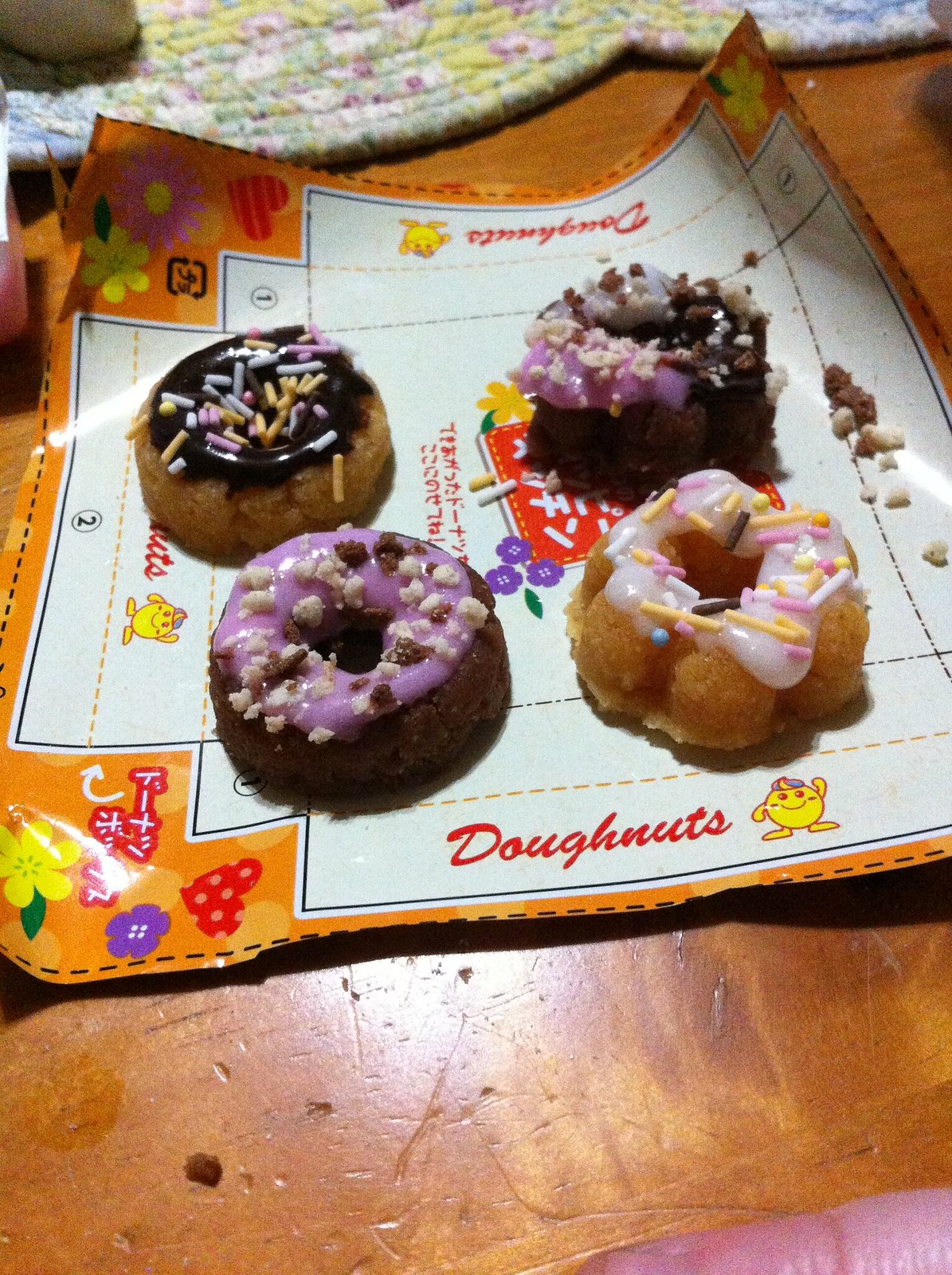This image showcases four mini donuts arranged on what appears to be a cutout placemat made from a flattened doughnut box. The placemat is colorful, featuring tangerine orange hues adorned with flowers, hearts, and a round yellow character with frosting on its head. The mat includes both Japanese katakana characters and the word "donuts" inscribed on each side except the right.

Each donut is uniquely decorated: two are chocolate and two are plain. All are topped with frosting and sprinkles. One chocolate donut features pink and white icing, while the other has purple icing with chocolate and vanilla crumbs. One of the plain donuts is topped with white frosting and decorated with yellow, pink, and white chocolate sprinkles. The final donut, positioned at the forefront, resembles a flower or Bundt cake, is plain, and has purple, brown, and blue icing.

In the background, there's evidence of a well-worn wooden floor and possibly a person or furniture element slightly out of focus. The placemat on which the donuts rest seems homemade, suggesting a personal, creative touch to the presentation.